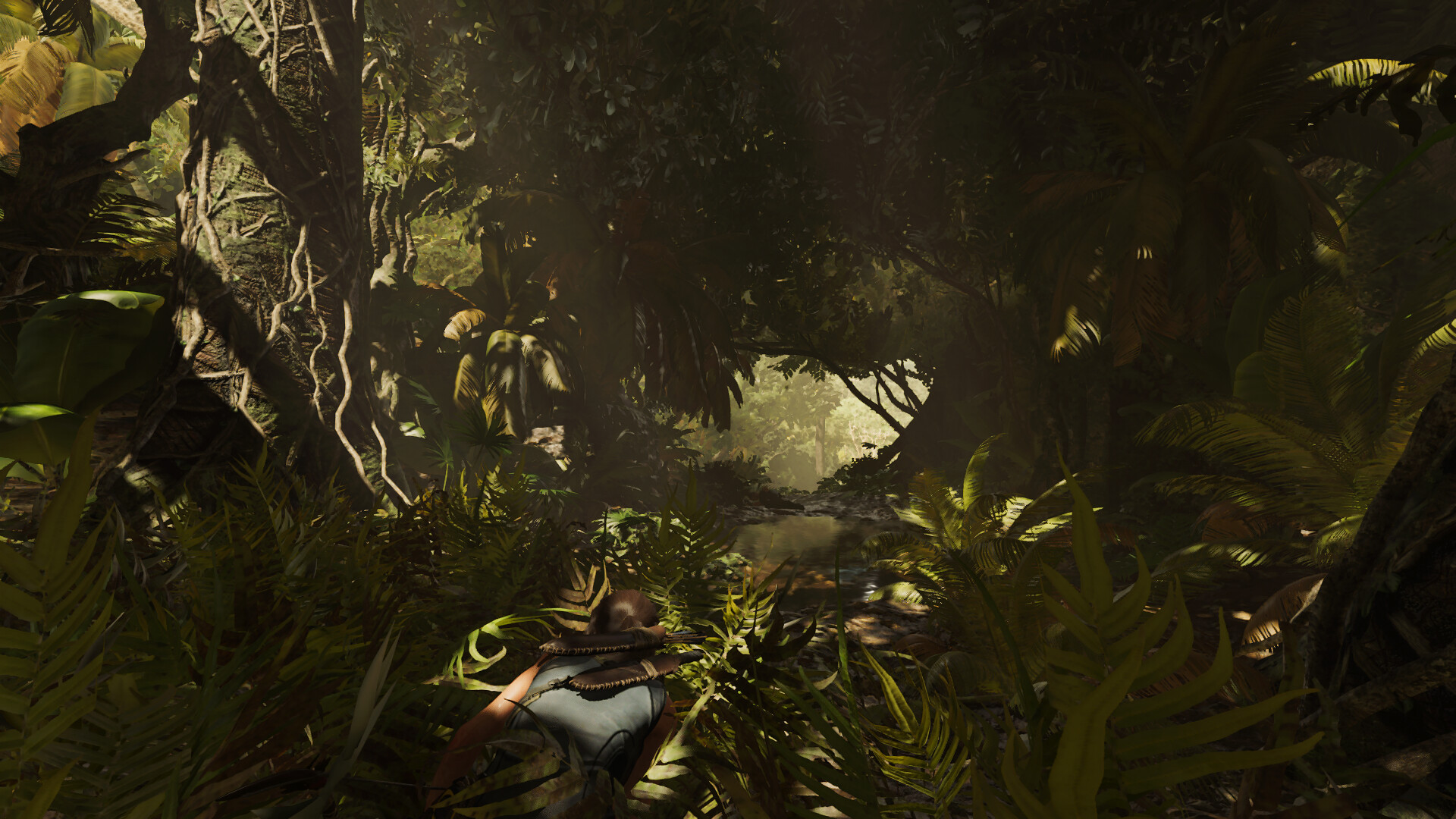The image portrays a highly detailed digital or AI-generated artwork depicting an incredibly dense, jungle-like forest. The scene is cloaked in deep shadows, almost forming a dark tunnel composed of entangled vegetation, thick foliage, trees, and vines hanging down in scraggly strands. The jungle atmosphere is palpable with green hues suffusing the entire scene. In the center of this lush, secluded environment, a small, nearly circular opening allows sunlight to pour through the canopy, casting a bright, concentrated beam of light. This beam illuminates the lower part of the image, reflecting off what appears to be a small body of water. Partial glimpses of human limbs—a pair of legs clad in blue pants and an arm—are subtly visible at the bottom of the frame, hinting at a human presence. On the right side, the tree line ascends and curves over the illuminated patch, adding depth and framing the bright focal point. The overall effect creates a striking contrast between the impenetrable darkness and the piercing light, evoking a sense of mystery and exploration within a hidden, jungle retreat.